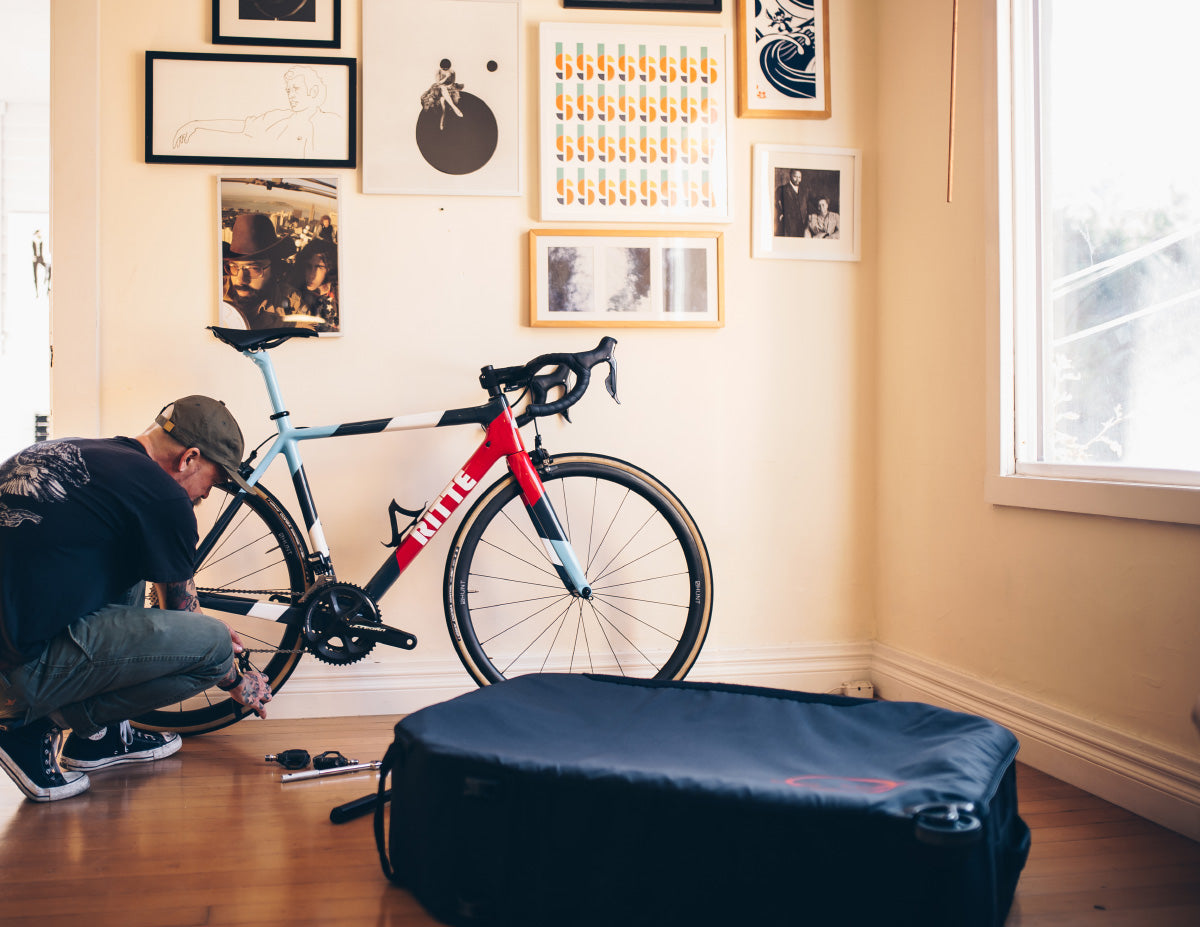In this detailed photograph, a man is crouched down inside what appears to be a warmly lit apartment or house, meticulously working on a bicycle chain. He is dressed in a black shirt, blue jeans, and black shoes with white soles, and he sports a dark brown baseball hat. The bicycle he is focused on is an eye-catching mix of light blue, black, white, and red. Surrounding him, the scene provides a cozy, lived-in feel with dark brown hardwood floors and cream-colored walls adorned with various paintings and portraits. A large window to the right allows natural light to stream in, illuminating the room. At the bottom center of the image, there's a large black suitcase with visible wheels and a red symbol, though its full design is obscured by the angle. Scattered around the man are several tools, indicating a workspace dedicated to his repair efforts.